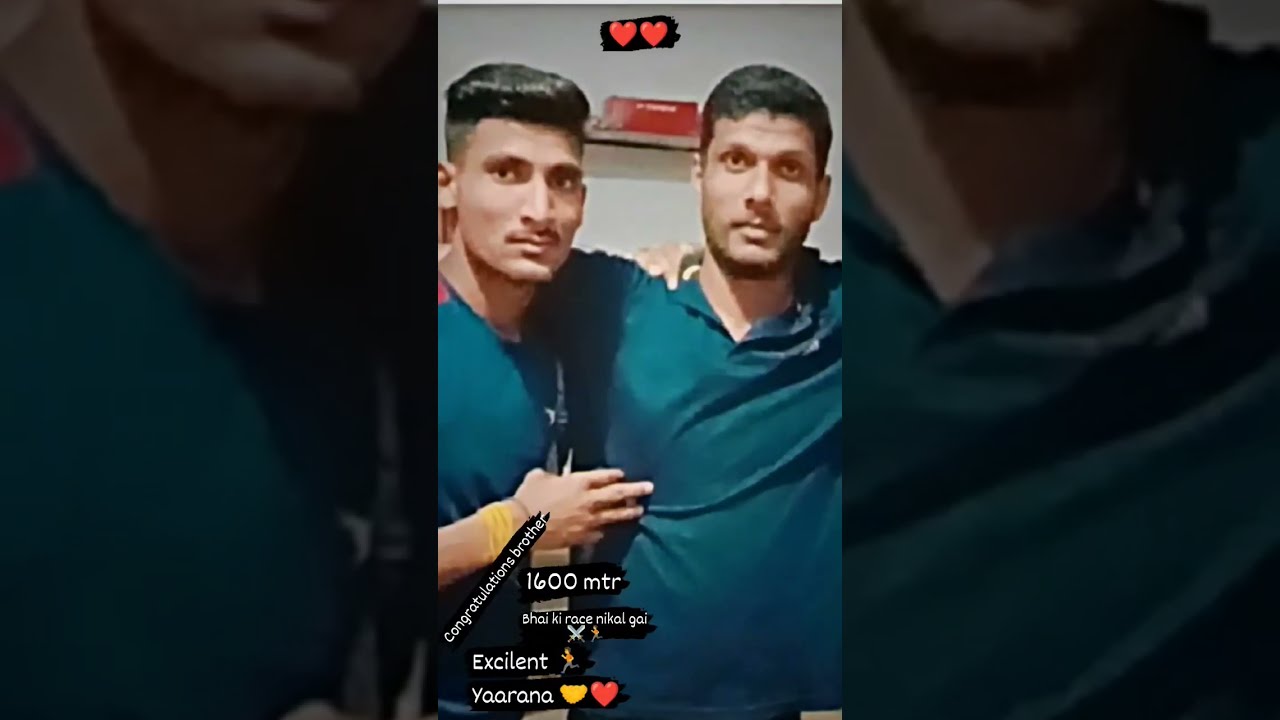The image is divided into three equal sections, with the outer sections in black and the central section featuring a photograph of two men. These two men, who appear to be Middle Eastern or Indian based on their skin color, stand closely together with their arms affectionately wrapped around each other's shoulders. Each man is wearing a sea blue or teal shirt, though one has a polo style and the other a T-shirt. The man on the left has slicked-back hair with shaved sides, a small mustache, and his right hand touching the chest of the man on the right, who has short, natural-looking hair and stubble. Above their heads are two red, animated hearts atop a black brushstroke, suggesting their close bond. Overlaid in the bottom corner of the image are celebratory banners with text saying, "Congratulations Brothers," "1600 meters," "Ba Ki Reis Nai Kal Gai," "Excellent," and "Yarana." The styles of the text and layout suggest that the image is from a social media page or website, celebrating the men's achievements, possibly in athletics.